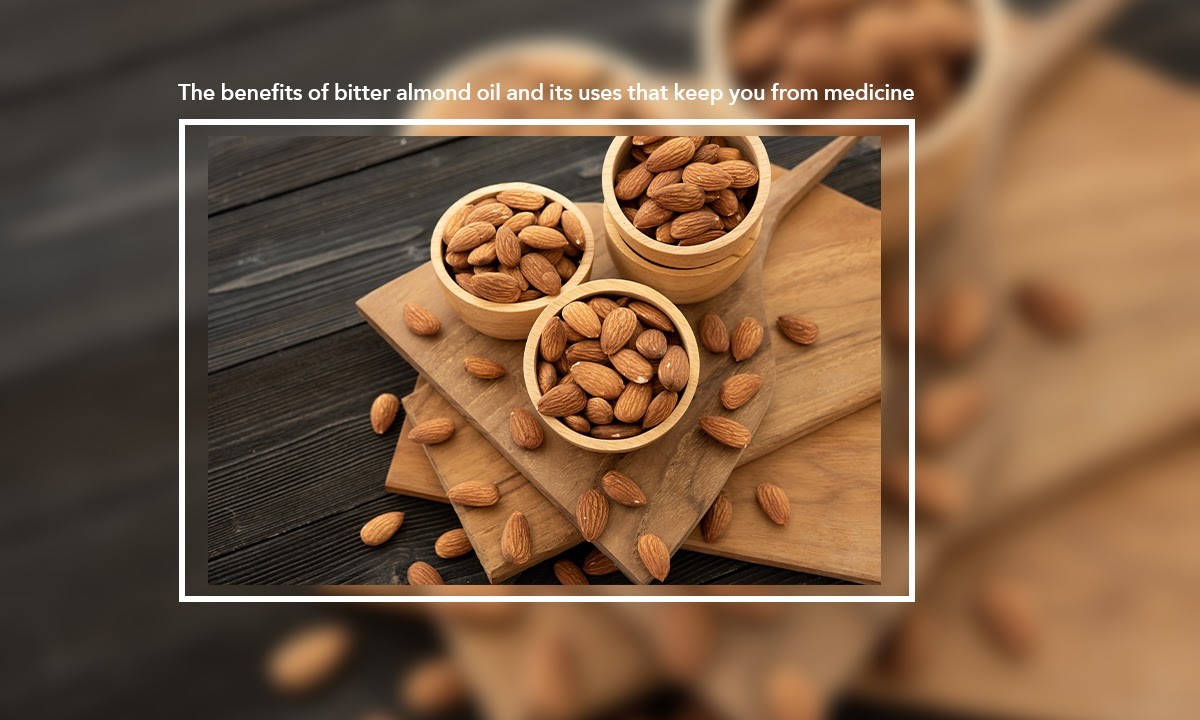This detailed image showcases a composition centered around fresh almonds and their health benefits. Positioned on a dark gray wood surface, there are multiple wooden cutting boards, each adorned with neatly arranged and scattered almonds. In the focal point of the scene, three bowls brimming with almonds are clearly visible, with another bowl partially nesting inside one of them, making a total of four. An additional utensil, resembling a spatula, adds to the rustic arrangement. The entire setup is encased in a rectangular photograph that is superimposed over a larger, blurred version of the same image, creating a layered effect. The clear, central photograph is framed with a white border and bears a prominent caption at the top that reads: "The benefits of bitter almond oil and its uses that keep you from medicine." This emphasizes the health advocacy aspect of the image, suggesting that bitter almond oil can serve as a beneficial alternative to traditional medicine.